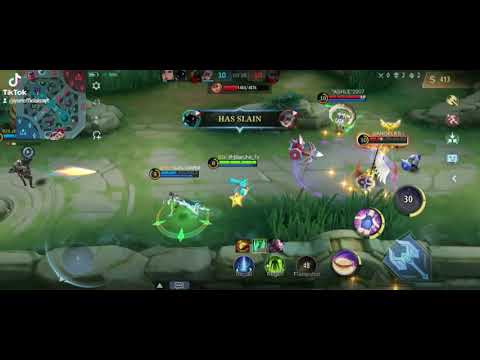The image is a low-quality screenshot of a video game, likely an action or role-playing game, captured from TikTok, as indicated by the emblem in the upper left corner. The screen is bordered by black letterbox bars at the top and bottom. The main game scene depicts an overhead view of a grassy field with gray stone pathways. Various indistinct characters populate the field, seemingly engaged in a battle, with magic powers in use, evidenced by yellow sparkles and a silver arrow bow. A message reading "has slain" suggests a recent in-game kill. In the lower right corner, circular controls are visible, including one resembling a large axe. Additionally, a small dark figure can be seen on the left side of the screen, while towards the right center, some angel-like characters appear. The mini-map is also visible in the upper left corner, contributing to the details on the screen.